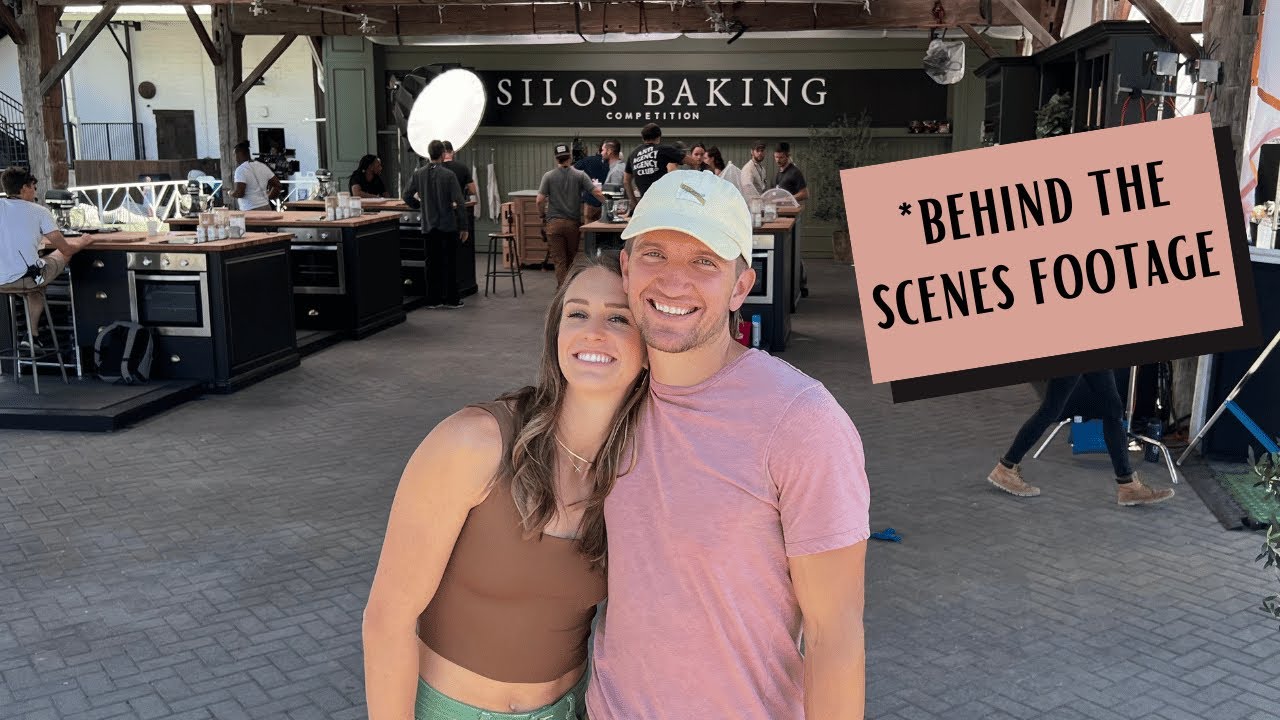This photograph captures a behind-the-scenes moment at the "Silos Baking Competition," as indicated by the black sign with white lettering visible in the background. Prominently featured in the foreground are a man and a woman, both fair-skinned and approximately in their 30s, who are smiling brightly and hugging. The man's exceptionally white teeth catch the eye, and he is dressed in a pink shirt with a white ball cap, while the woman wears a brown tank top and green pants. The image cuts them off at the waist. The floor beneath them is made of cement or patio bricks, arranged in a diagonal tile pattern. In the background, various baking stations are set up, complete with ovens and preparation tables, where people are either sitting or engaged in different activities, possibly taking a break. The scene is brightly lit with several lights and cameramen visible, contributing to the detailed clarity of the photo. A pink box on the right-hand side of the image includes an asterisk and the text "behind-the-scenes footage," reinforcing the notion that this is a candid glimpse into the workings of a reality baking competition show.